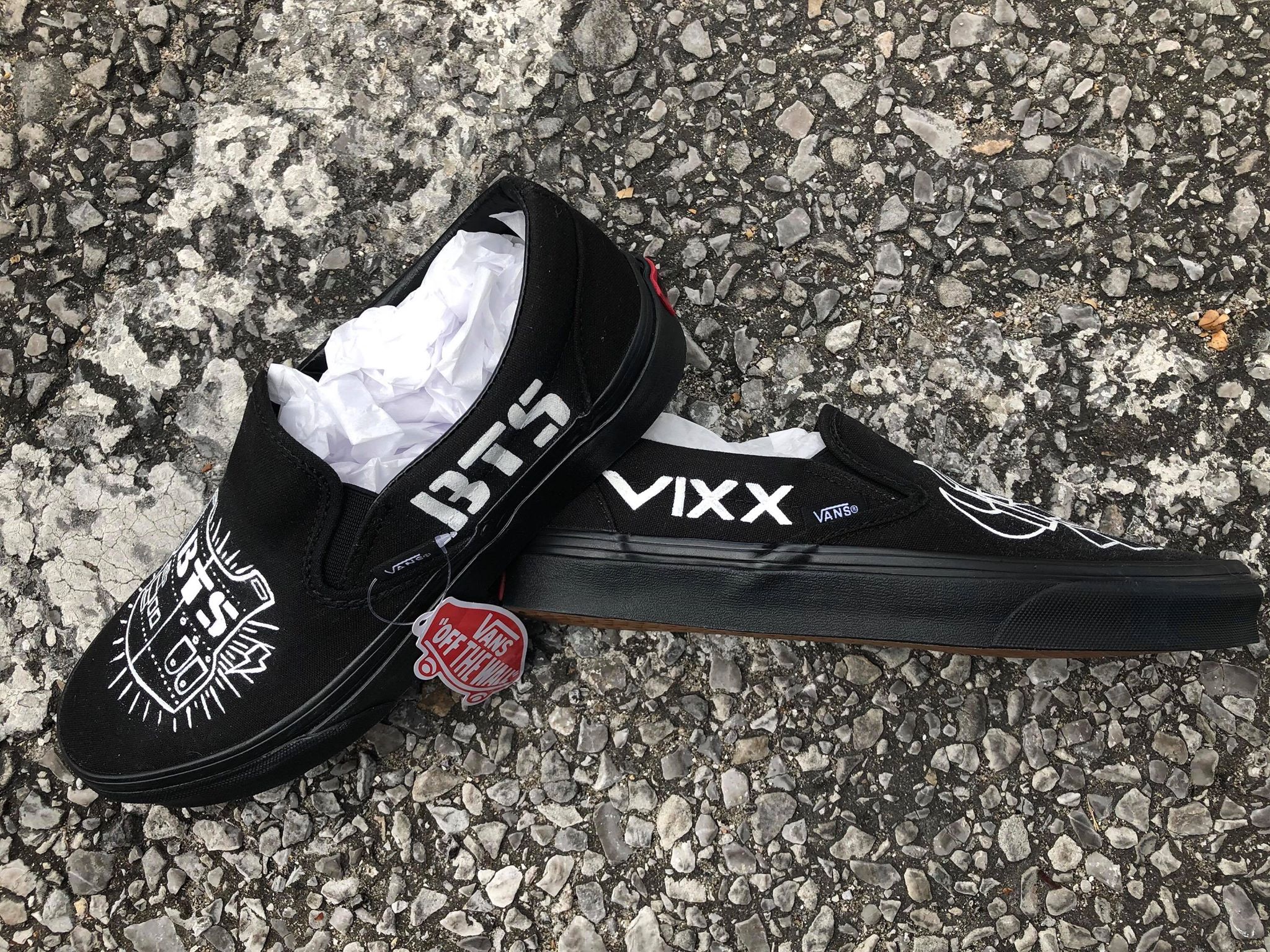This color photo captures a pair of black Vans slip-on sneakers laying on a textured asphalt road scattered with small rocks. One shoe lies on its side facing right with the word "VIXX" in white, while the other is propped up on the first shoe facing left, displaying the word "BTS" in white on the side. The left shoe also features a distinctive white shield-like design on the top, adorned with the letters "BTS" and embellished with lightning bolts and rays. Both shoes are tagged with the Vans logo; the left shoe features a prominent red tag with the phrase "Vans Off the Wall." The interior of each shoe is visibly stuffed with crumbled white paper, suggesting they are brand new and possibly set up for an advertisement.